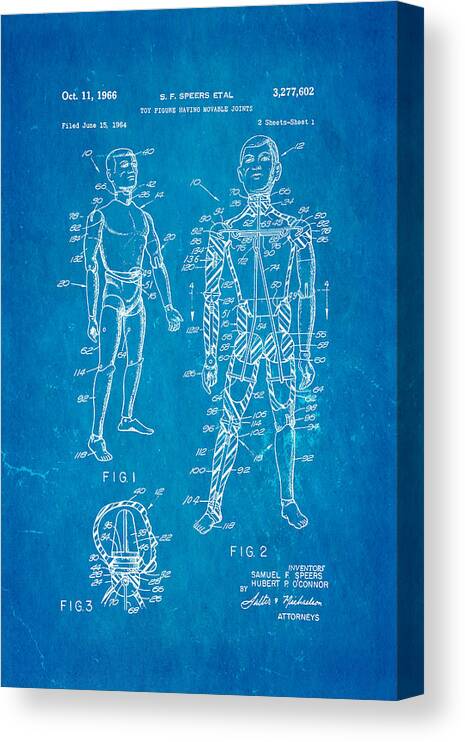The image portrays a vertically rectangular, blue display resembling a scientific poster or a patent illustration, with a three-dimensional appearance visible from the spine on the right edge. The background is uniformly blue, and the poster is extensively detailed with white diagrams and annotations.

The display features three primary figures related to human anatomy:
1. Figure 1 depicts a human body facing right, with various numbers and lines pointing to different anatomical areas around the heels, shins, and joints.
2. Figure 2 is a larger, frontal view of a human body, subdivided into sections with even more detailed annotations and lines indicating specific points on the body.
3. Figure 3 presents a side view of a human head, similarly annotated with lines pointing to significant areas.

In the upper left corner, the poster is dated October 11, 1966, and there’s a filing date of June 15, 1964. Above the figures, the number 3,277,602 is prominently displayed. Additionally, the names S.F. Spears and others (not fully distinguishable) are listed, likely representing those involved in the creation of the diagram. Further down, names such as Sammy Hubert and Spears are written alongside the term "Attorneys," possibly indicating the individuals responsible for filing or authorship.

Overall, the poster serves as a detailed anatomical chart with precise annotations, presenting a combination of dates, names, and figures indicative of a scientific or patent-related document.